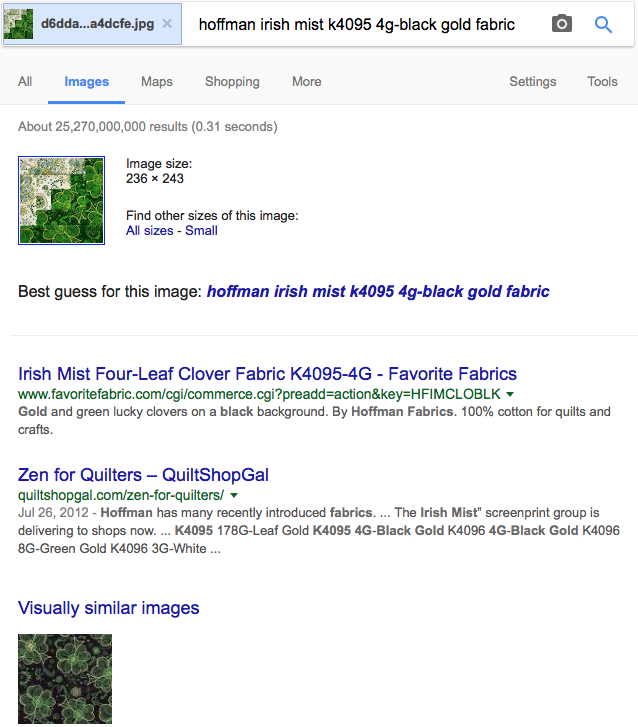**Image Description: Detailed Search Results Page**

The webpage depicted shows search results, presumably for an image search. At the top, there's a small blue bar featuring a square icon in the upper left corner. This icon contains a white design and a green, stair-like pattern at the bottom right corner, labeled as a ".jpg" file with random letters and numbers.

To the right of the icon, there's a white search bar displaying the text: "Hoffman Irish mist k4095k 4g dash black gold fabric." Adjacent to the search bar are camera and search icons. Below this, a navigation bar offers typical Google options: "All," "Images," "Maps," "Shopping," "More," and "Tools." The "Images" option is selected, highlighted in blue with an underline.

Beneath the navigation bar, search results indicate around "25,270,000,000 results (0.31 seconds)." The first result features the same green and white symbol, stating "Image size: 236 by 243." It offers the option to "Find other sizes of this image," followed by clickable links labeled "All sizes - small." The best guess for the image's contents is listed in blue text as "Hoffman Irish mist k4095k 4g dash black gold fabric."

Two primary website results follow. The first link, titled "Irish Mist Four-Leaf Clover," leads to "www.favoritefabric.com." It describes the image as "Golden green lucky clovers on a black background by Hoffman fabrics, 100% cotton, for quilts and crafts." The second result, "Zen for Quilters - Quilt Shop Gal," links to "quiltshopgal.com," dated July 26, 2012, and provides additional details about the same fabric.

At the bottom of the results, a section titled "Visually similar images" is shown in blue, accompanied by an image of four-leaf clovers on a black background.